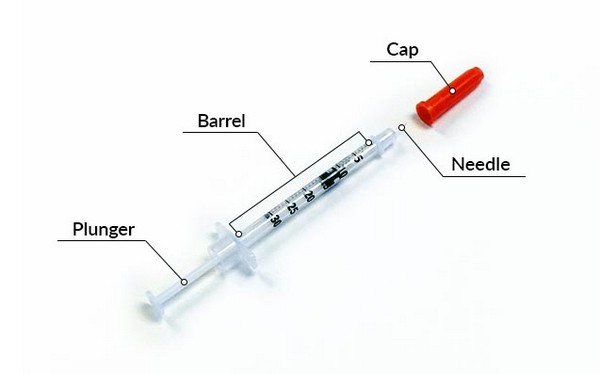The image depicts a detailed diagram of a disassembled syringe against a stark white background. The syringe components are laid out diagonally, with the clear tube and needle extending from the bottom left towards the center, and the dark orange-red cap resting at the top right. Each part of the syringe—the cap, needle, barrel, and plunger—is meticulously labeled with connecting lines and descriptions. The barrel, which is transparent, features numerical markings ranging from 5 to 30, allowing visibility of the stopper inside. Shadows cast by the syringe parts suggest a slight three-dimensional effect, enhancing the clarity of the educational diagram. The overall presentation indicates an instructional setting, aimed at teaching the anatomy and usage of a syringe.